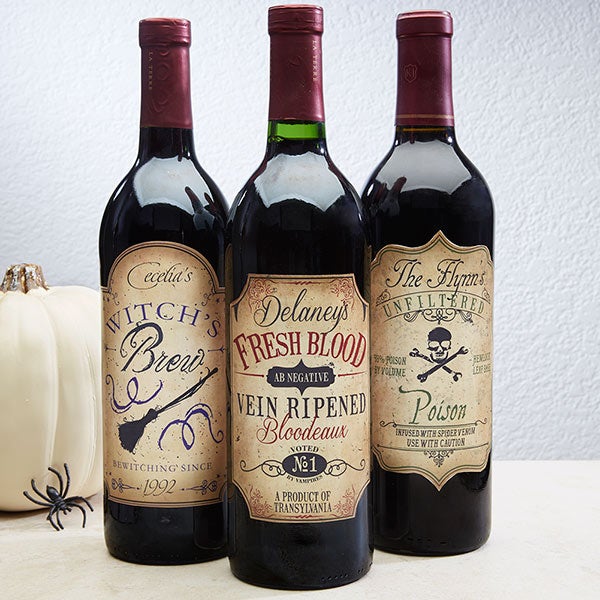This image showcases three dark bottles of red wine, each with a distinctive tan label, arranged on a white tablecloth. The background is a textured white wall, enhancing the overall contrast. To the left of the frame, there is a decorative white pumpkin with a gold stem, accompanied by a small black plastic spider ring in front of it. 

The first bottle on the left is labeled "Cecilia's Witches Brew," featuring an illustration of a broom and the phrase "Bewitching since 1992." 

The middle bottle is called "Delaney's Fresh Blood" with additional text in red stating "Vain Ripened Bordeaux" and "a product of Transylvania."

The bottle on the right is labeled "The Flynn's Unfiltered" adorned with a pirate skull and crossbones, and the word "Poison" in green text underneath.

Each bottle is sealed with a deep burgundy-red wax, adding to the mysterious and festive ambiance of the display.